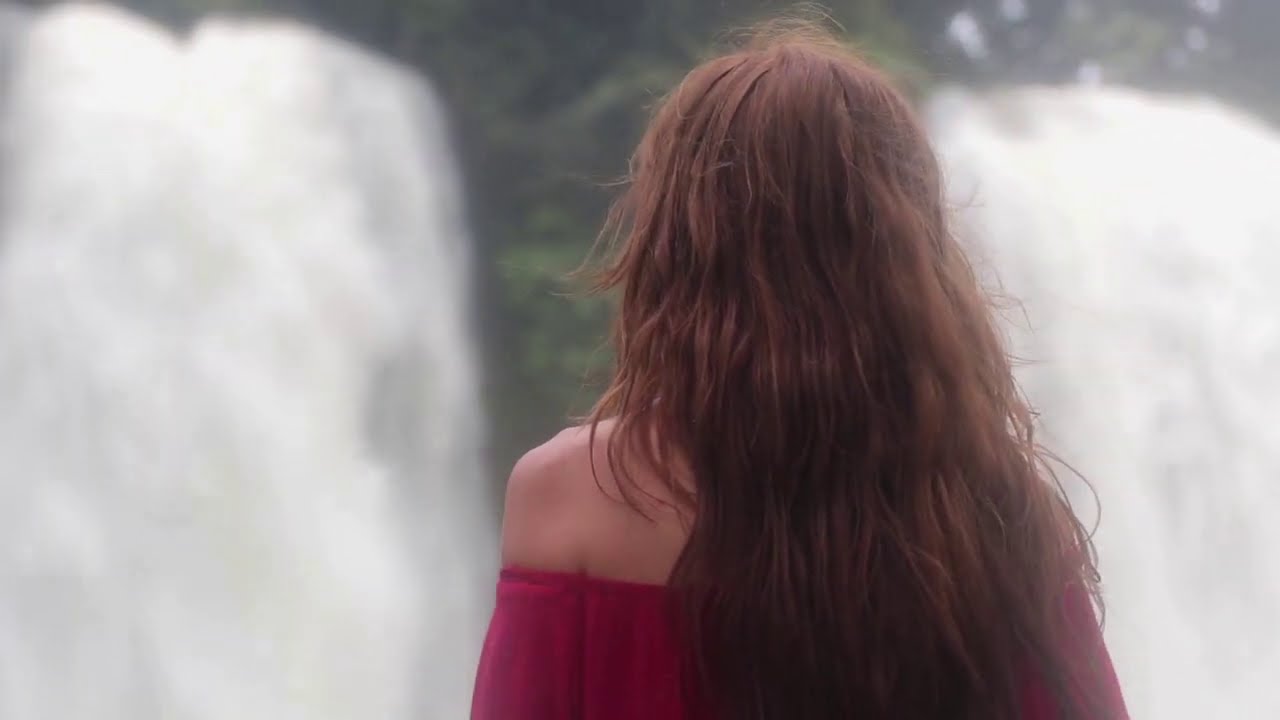This photograph captures the back of a woman with long, dark red or brown hair that reaches the middle of her back. She is wearing a red or maroon top that leaves her shoulders bare and falls to mid-upper arm. She stands outdoors in the daytime, with no indication of strong wind as her hair is not windswept. The background is blurred but features two bright white waterfalls cascading down on either side of her, separated by a section of lush greenery on the hill from which the waterfalls flow. Although the waterfalls and the landscape behind her are blurry, the photograph highlights the serene and natural environment she is observing.